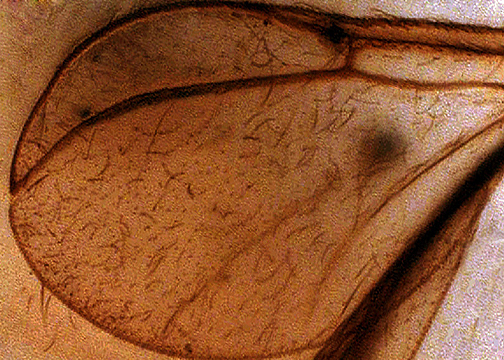This detailed image reveals a close-up view that appears to have been taken under a microscope. Dominating the center is a structure with noticeable layers and a prominent line running through its middle. There's a black spot on the right side, casting a shadow beneath it. The texture of the structure is intricate, featuring tiny hair-like filaments, some of which are black and brown. The overall coloration shifts from a light tan on the left side to a mix of wider tannish and gray hues toward the top and bottom right corners. The surface resembles skin, potentially highlighting a tattoo, with distinct outlines and gradients of color. The intricate pattern of hairs and the layered structure suggest this could be the highly magnified wing of an insect, such as a moth or butterfly, further emphasized by the microscopic perspective.